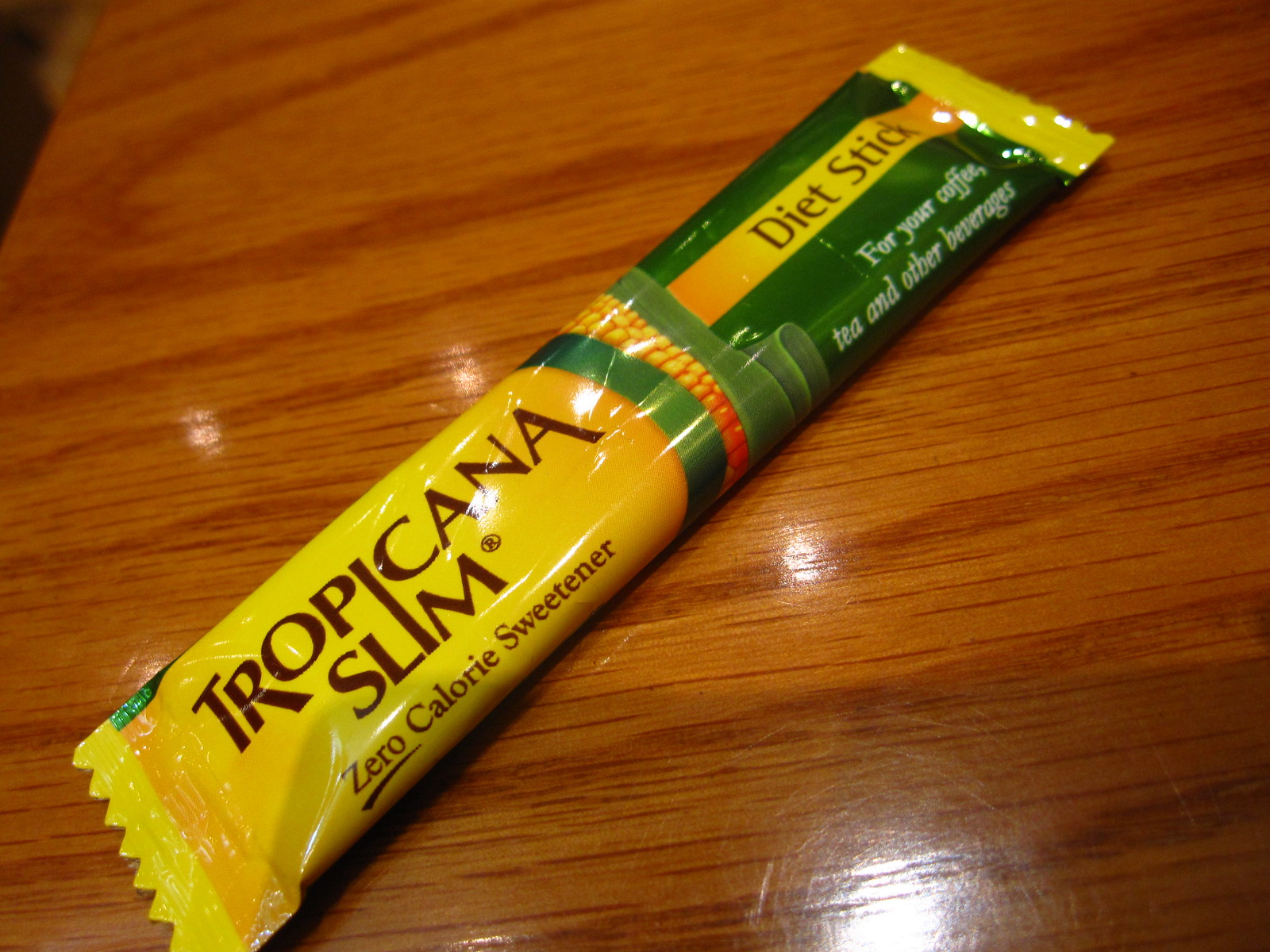This is a detailed color photograph of a long, slim packet of sweetener, prominently featuring the brand Tropicana Slim. The packet, primarily yellow on the left and transitioning to green on the right, is emblazoned with brown letters that read "Tropicana Slim zero calorie sweetener," with "Zero" notably underlined. Additionally, the packet conveys in white text, "Diet Stick for your coffee, tea, and other beverages." A partially visible image of a corn cob is situated near the center of the design. The packet lies diagonally on a light-colored wooden table, extending from the bottom left corner towards the upper right. The photograph, likely taken with a personal camera or cell phone, captures light reflections both on the packet and on the wooden surface. No people, animals, plants, flowers, trees, or motorized vehicles are present in this image.